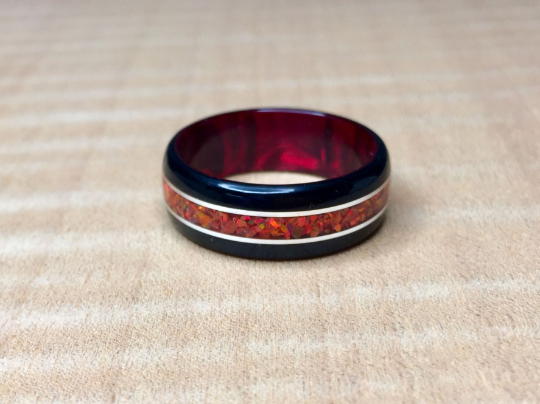This close-up image showcases a detailed ring, likely designed as a wedding band, crafted to demonstrate the jeweler's intricate work. The ring exhibits a sophisticated pattern of alternating stripes: starting with a dark band on top, followed by a very thin white band, then a thicker orange speckled stone band in the middle, another thin white band, and finishing with a dark band at the bottom. The vantage point of the photo is slightly above the ring, allowing a view of both its outer and inner surfaces. Notably, the inner surface appears to have a transparent dark red hue when illuminated by sunlight, suggesting it might be made of resin or acrylic. The ring is placed on a tan and white cloth background, enhancing its distinct color contrasts and detailed craftsmanship.